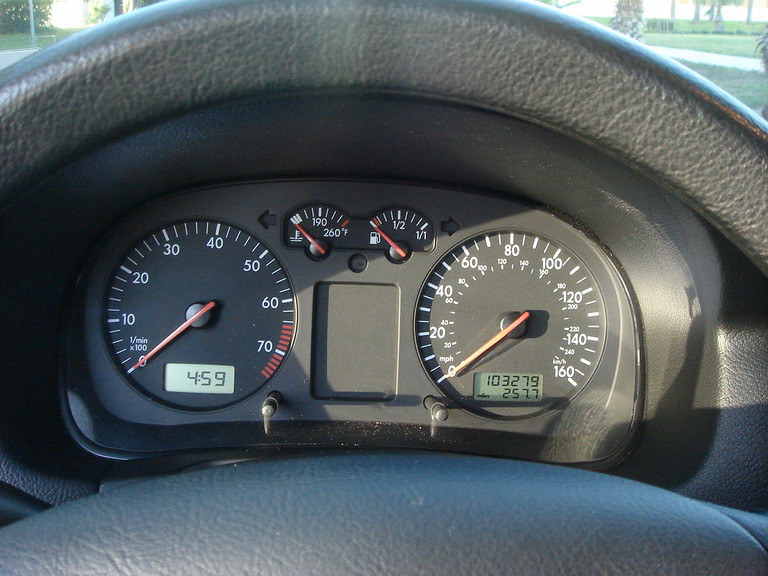The image captures the interior of a car from the perspective of the driver's seat, showcasing the dashboard and its various instruments. In the center of the dashboard, behind the steering wheel, multiple dials and indicators are visible.

To the left, there is a circular gauge with numerical markings from 10 to 70, increasing in increments of ten. This gauge also displays the time, showing "4:59." 

In the middle of the dashboard, two smaller indicators can be seen. The one on the left likely represents the temperature, while the one on the right indicates the fuel level, which appears to be nearly empty as indicated by the red pointer.

On the far right, there is a larger speedometer that measures speed from 20 to 160 miles per hour, increasing in increments of twenty. Below this, the odometer displays a reading of 103,279 miles. The dashboard layout is detailed with each element precisely marked, giving a comprehensive view of the car's operational status.